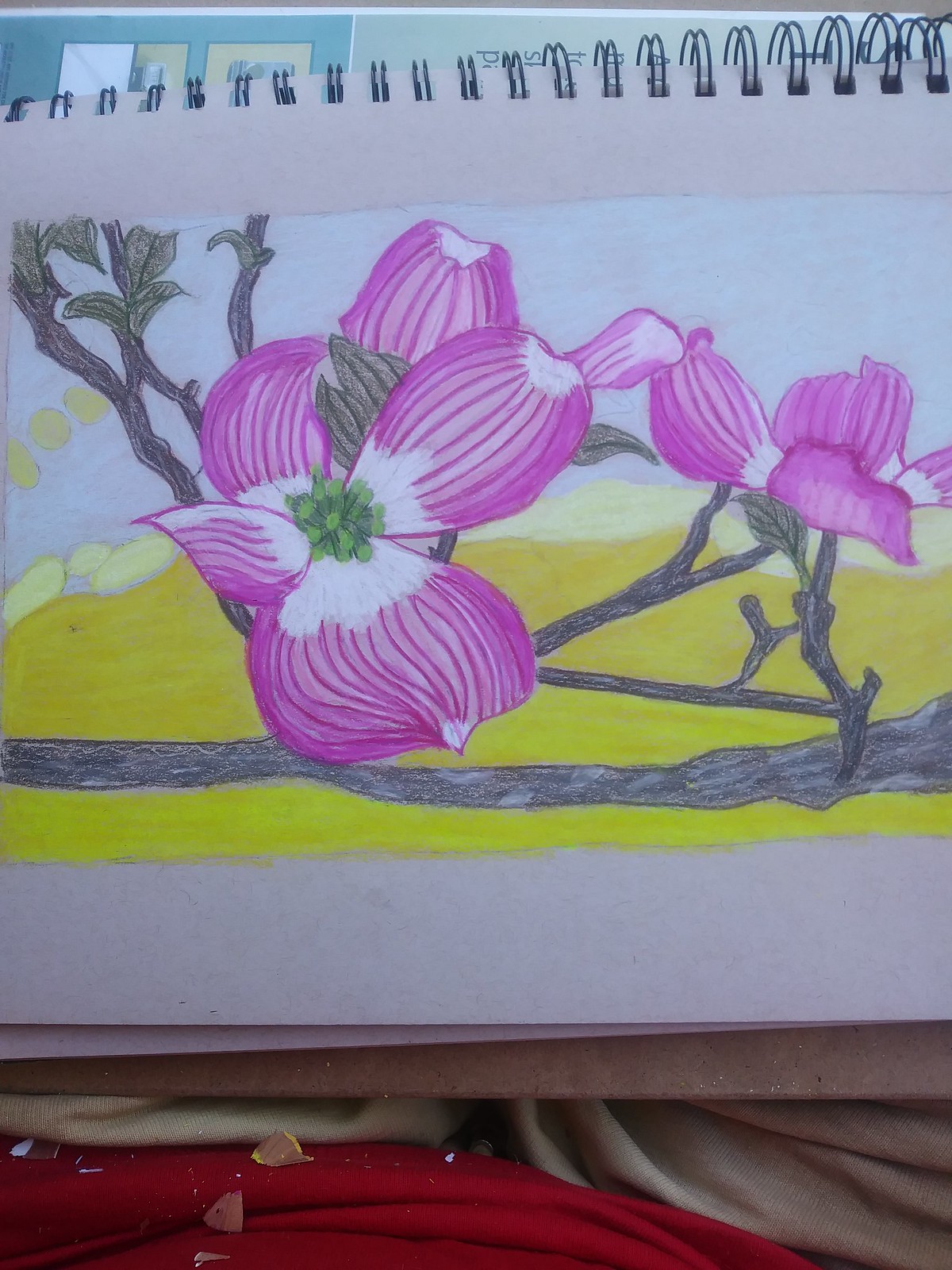The image depicts a detailed watercolor painting of Japanese cherry blossom flowers in a drawing sketch pad. The blossoms are primarily pink with some white accents and a green center. They are situated along horizontal brown branches that have a few green leaves sprouting from them. The background features a blend of yellow, white, and blue shades, giving it a soft and layered appearance. At the top and side of the image, the metal spirals of the sketch pad are visible, indicating that the painting is done on spiral-bound paper. The entire sketch pad rests on someone's lap, where the person's red shirt and tan pants are discernible. Additionally, there are some pencil shavings scattered on the shirt, and the whole setup is supported by a brown cardboard base.